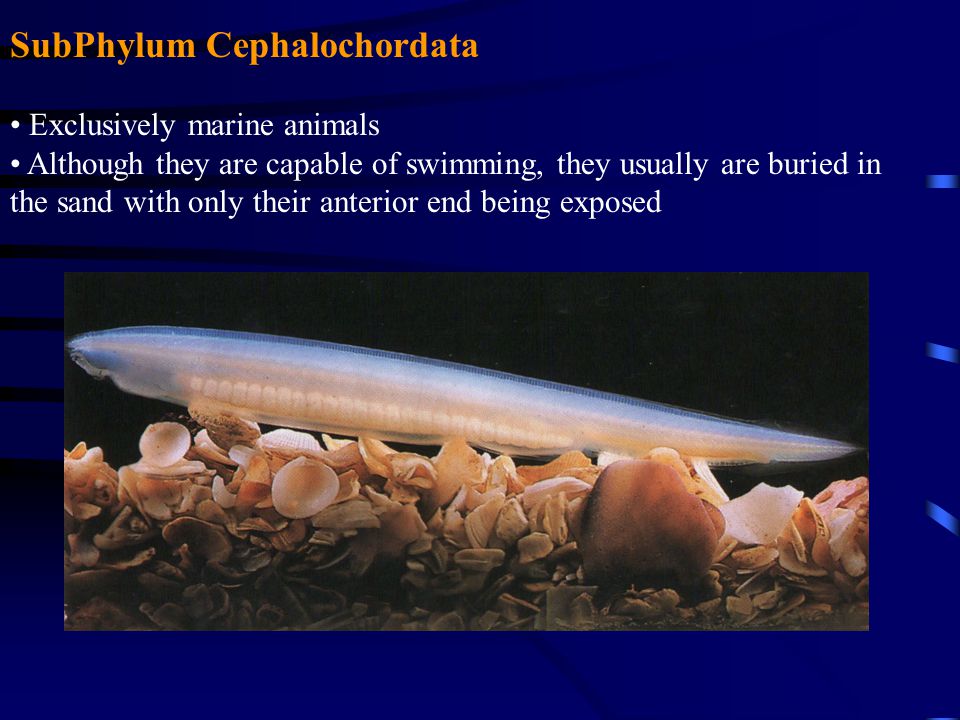The image features an informative slide about marine animals titled "Subphylum Cephalocordata." The overall background is a dark blue, providing a stark contrast with the colorful text. At the top of the slide, the title "Subphylum Cephalocordata" is prominently displayed in yellow text, with the description "Exclusively marine animals. Although they are capable of swimming, they usually are buried in the sand with only their anterior end being exposed" written below in white. 

The bottom portion of the slide illustrates a specific marine animal, which is a tiny, translucent fish-like creature. This creature appears to be situated deep underwater, indicated by the darkness of the surrounding environment. The animal's body is elongated, mostly clear with a visible spinal structure, and it tapers to a sharp point at the anterior end. Surrounding the creature are seashells and sediment, adding to the natural underwater scene. The colors visible in the image include shades of blue, orange, white, silver, gray, brown, and tan, emphasizing the vivid detail and clarity of the illustration on the slide.